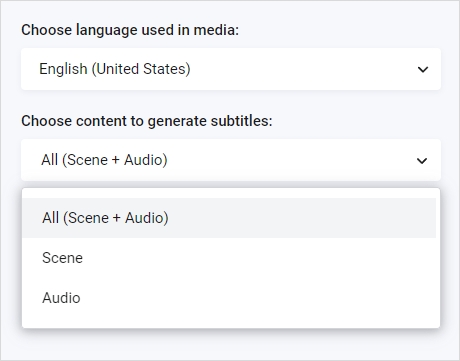The image displays a light gray background with a slightly darker border along the perimeter. In the top left corner, in nearly black text, it reads "Choose Language Used in Media:" with a capitalized "C." Below this text is a white rectangle containing the word "English" with the notation "(United States)," where the "E," "U," and "S" are capitalized. To the right of this text box is a drop-down arrow.

Further down, the image includes the instruction "Choose Content to Generate Subtitles:" also with a capitalized "C." Beneath this instruction is another white menu displaying the word "All" with a capital "A," followed by the phrase "(Scene + Audio)" where both "S" and "A" are capitalized. A drop-down arrow is positioned on the right of this menu.

Below this section is a lighter-colored rectangle with a highlighted banner overlaying the options "All (Scene + Audio)," "Scene," and "Audio." The option "All (Scene + Audio)" appears to be selected.